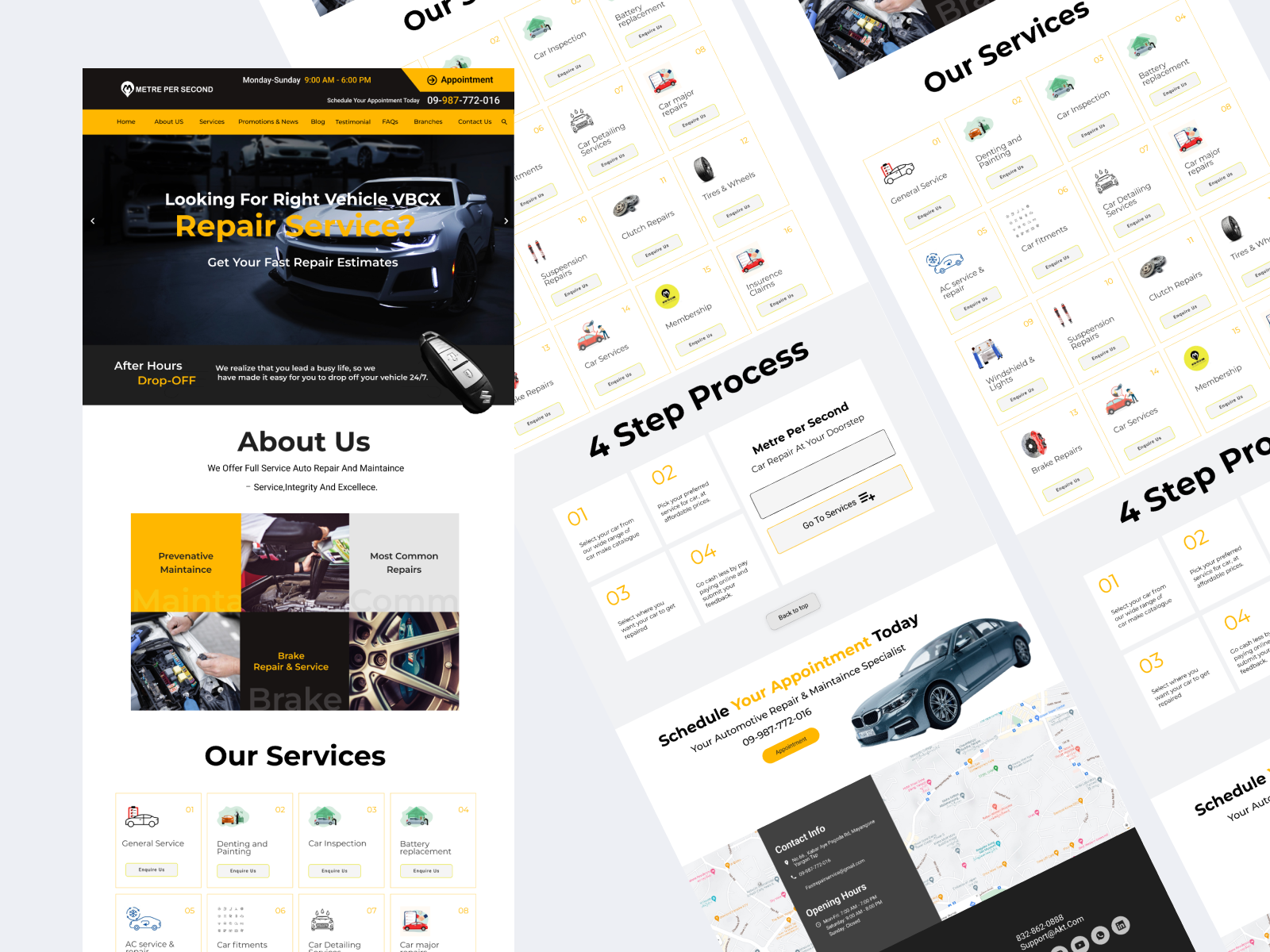Screenshot of an appointment scheduling interface for vehicle repairs. The screen prominently features the text "VBCX" in bold, uppercase letters. Below, there is a highlighted section in yellow that reads "Repair Service," encouraging users to get fast repair estimates. Additionally, the interface offers options for "After Hours Drop Off," "About Us," "Preventive Maintenance," "Brake Repair and Service," and lists "Most Common Repairs." There is a section labeled "Our Services" accompanied by thumbnail images, though these images are too small to discern clearly. On the right side, a multi-step process is described, detailing four steps involved in the repair service, each labeled with specific information. The term "meter per second" (abbreviated as "METRE") is also visible in this segment. The background of the interface is somewhat indistinct, providing a subtle backdrop to the detailed service options presented.